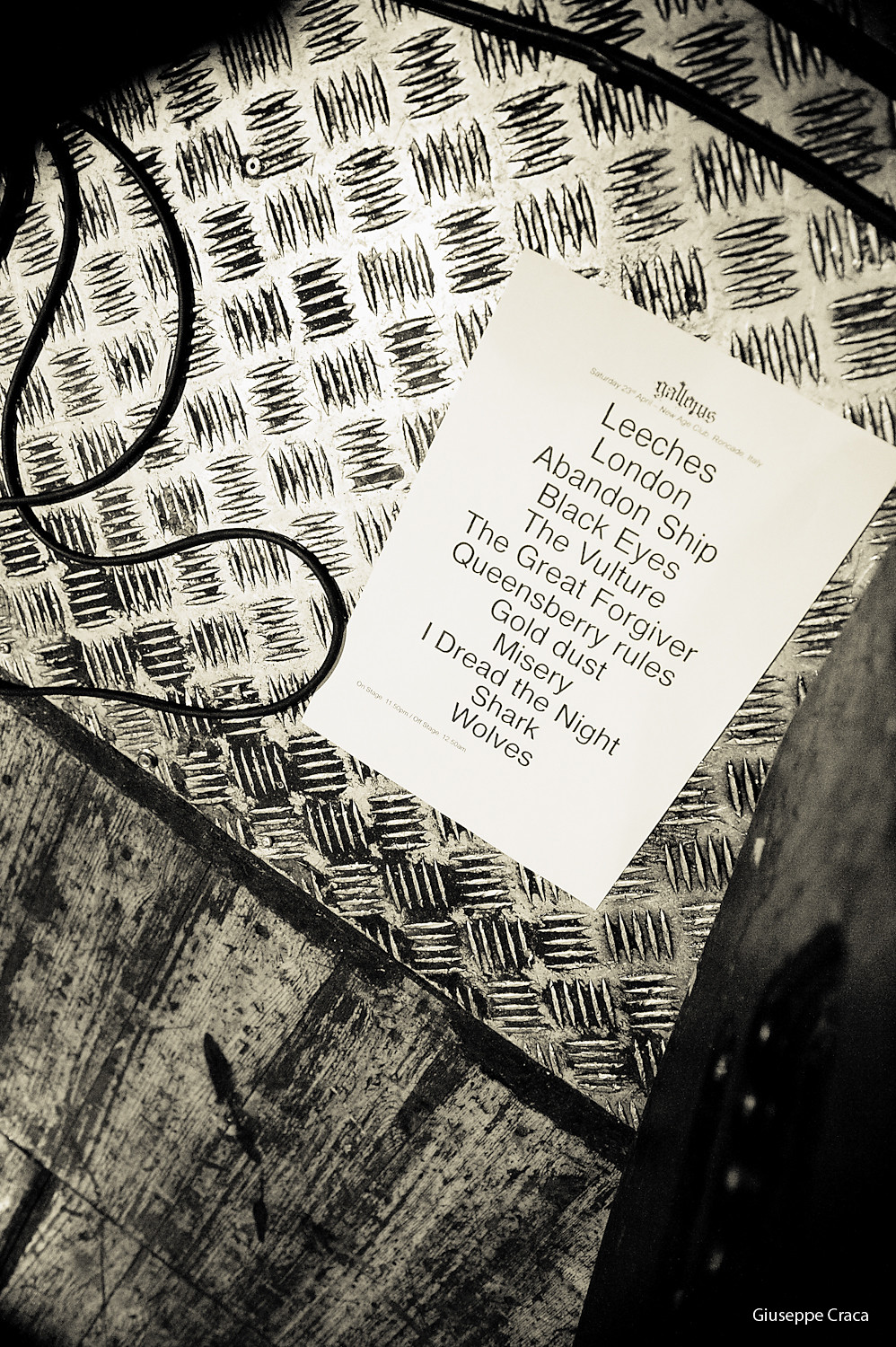This vertical rectangular black-and-white image features a detailed and complex background, giving a sense of an apron-like object with both intricate black-and-white patterns and possibly pockets or textured elements. Overlaying this backdrop is a piece of paper diagonally positioned, titled at the top (though the title is unreadable) and printed with a list of names in black ink. These names likely represent a set list of songs, and include: Leeches, London, Abandoned Ship, Black Eyes, The Vulture, The Great Forgiver, Queensberry Rules, Gold Dust, Misery, I Dread the Night, Shark, and Wolves.

In the upper right quadrant of the image, the names are prominently displayed on the white paper amidst the variegated background. The surrounding environment contributes an industrial or gritty feel, possibly hinting at a music venue where bands might perform, emphasized by surfaces resembling a metal grate and wood flooring. This fusion of elements creates a visually textured and evocative composition.